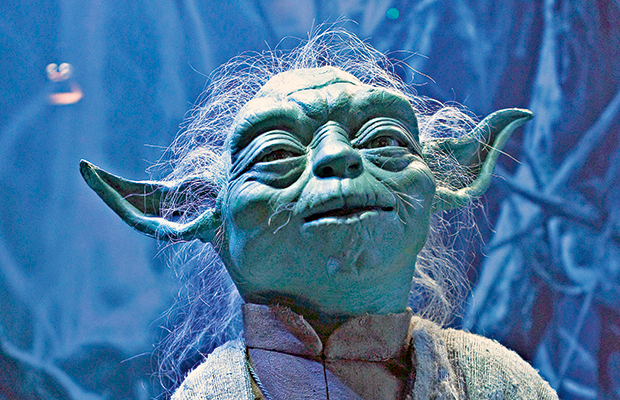The image depicts Yoda, the iconic character from the Star Wars franchise, captured in a close-up shot, facing the camera. Yoda has an aged appearance with a small, round head, heavily hooded eyes, and slightly parted lips, revealing no teeth. His skin is a light turquoise or aqua green hue, and thin, wispy white hair tufts stick out from his scalp. Distinctive long, pointy ears jut out from the sides of his head. He is clad in a high-collared, gray shirt topped with an off-white knit or crocheted cardigan. The background features a blurred, blue-toned sinuous forest scene with marred outlines of tall, sinewy vines and tree trunks, creating a murky, ethereal atmosphere. There's a light shining on Yoda's forehead and the tips of his ears, adding to the mystical ambiance of the image.